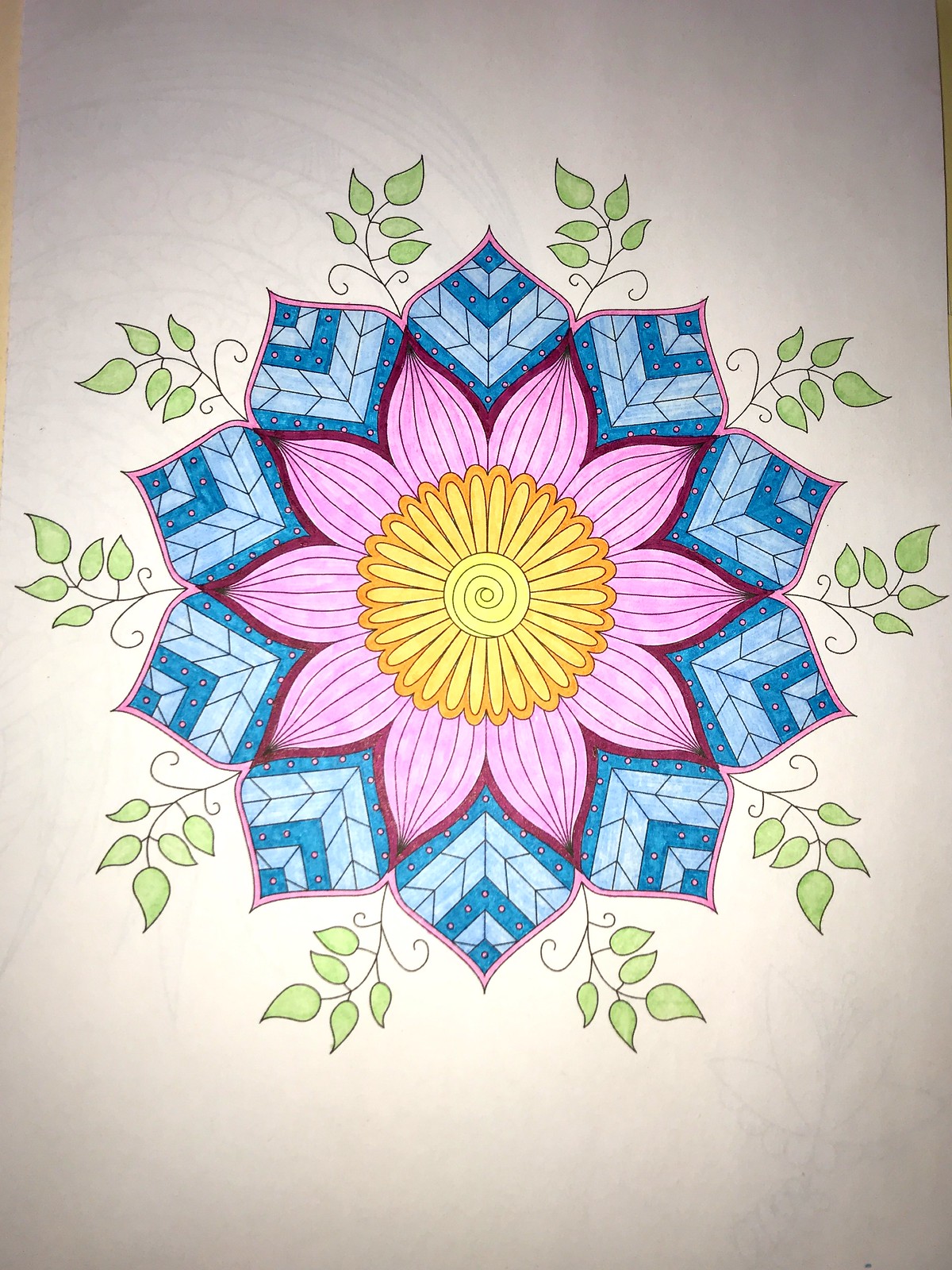This intricate hand-drawn artwork showcases a central star pattern executed with a combination of colored pencils and markers. At the heart of the design lies a detailed flower featuring a large, round center adorned with a mesmerizing spiral. Radiating outwards, the flower's petals expand gracefully before tapering to a narrow edge, creating a rhythmical balance around the circumference. The flower's petals are outlined vibrantly in orange, contrasting beautifully with the surrounding elements.

Encircling the flower are purple petals, each outlined in a deeper purple hue, adding depth and dimension to the composition. Every purple petal is defined by five or six lines that converge to create pointed tips, forming a harmonious and repetitive pattern. Additionally, between each of these main purple petals, delicately drawn lines extend outward and then curve back in to meet at another point, contributing to the geometric complexity and visual intrigue of the piece. This artwork, rich in detail and color, captures both precision and creativity, making the flower a striking focal point amidst a symphony of shapes and hues.